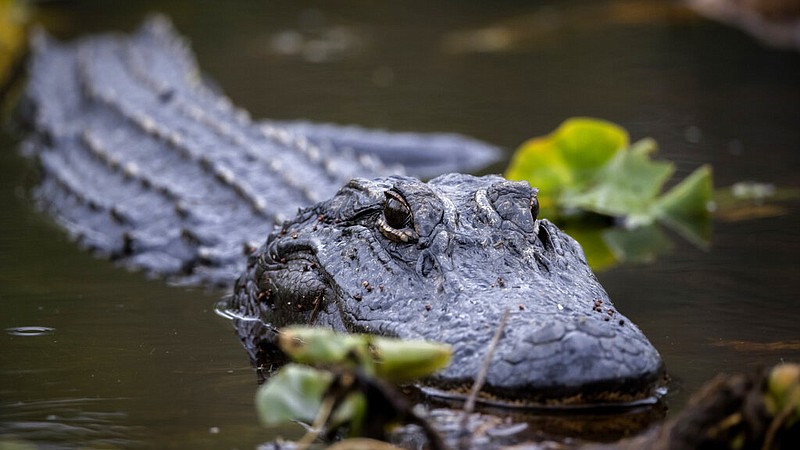In this detailed photograph, an alligator emerges from the swamp, its scaly body stretching diagonally from the upper left corner to the lower right corner of the frame. The creature's gray snout points towards the bottom right, while its black eyes dominate the middle of the image, with the right eye clearly visible. The body of the alligator fades out of focus as it extends upwards, and its tail appears to poke out above its head, again in the middle of the frame. The surrounding swamp water is a murky brownish-gray, dotted with floating leaf matter. Some leaves are green and black, gathered towards the bottom and middle right of the photograph. A brighter, slightly yellowish clump of leaves is positioned behind the alligator's head on the right side, blending into the background.